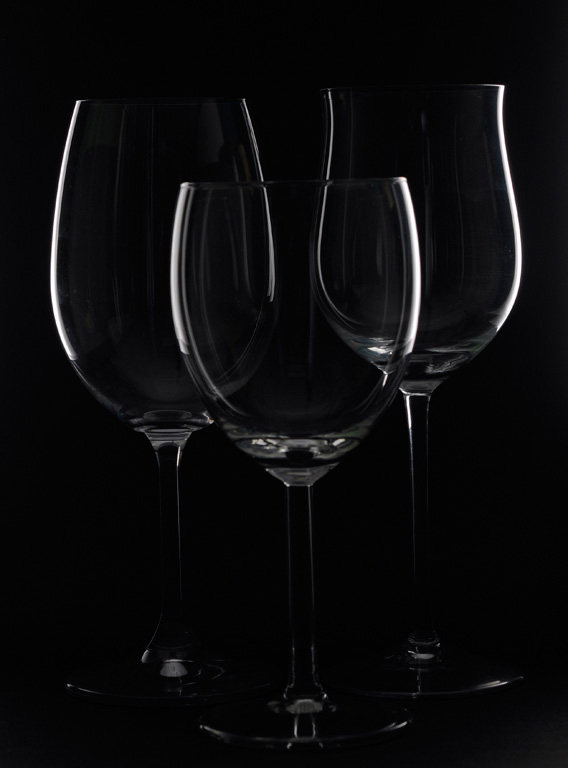This image is a striking photograph of three clear glass wine goblets, meticulously arranged in a triangular formation against a stark black background. The goblets are illuminated by subtle glints of light, revealing their delicate contours and making a dramatic visual impact. The goblet in the foreground is shorter and tulip-like, creating a focal point with its unique shape. Behind it, two taller goblets stand, similar in height but differing in design—the one on the left is a classic, more closed wine glass, while the one on the right features an elegant outward curve at the top. The uniform clarity and shininess of the glass emphasize the elegance and subtle distinctions in their forms, making the photograph both hypnotic and sophisticated.